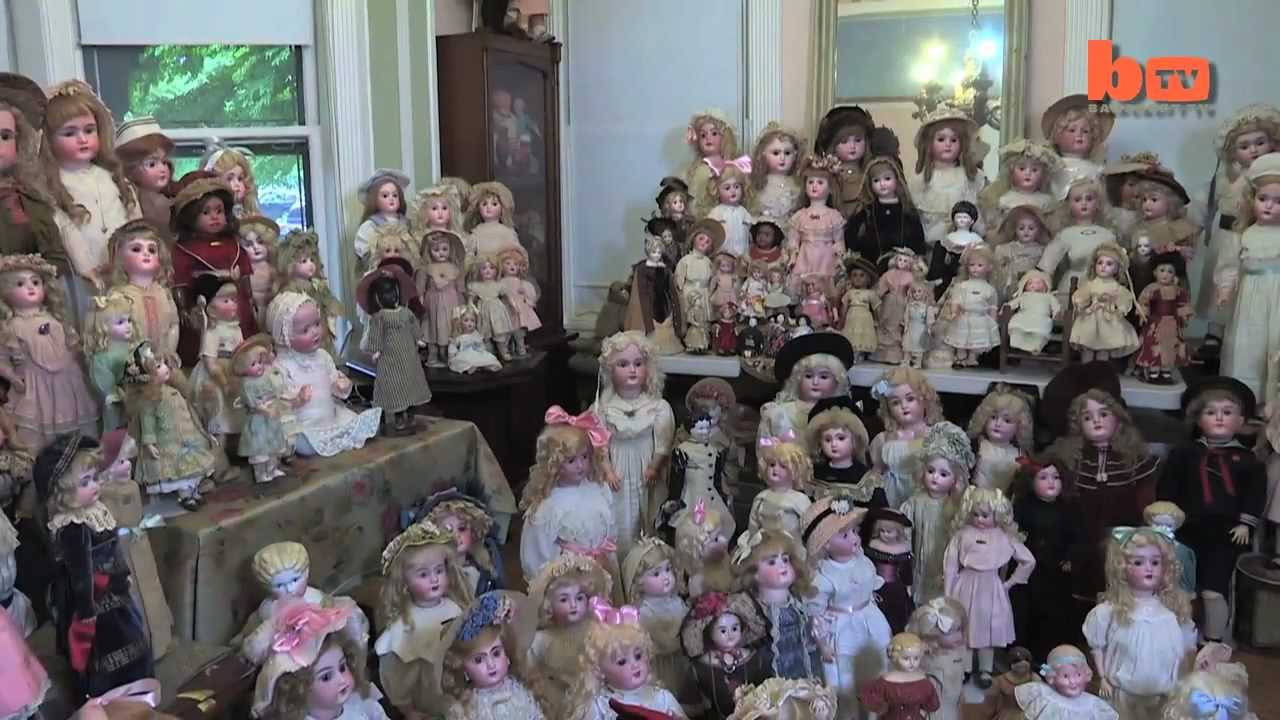The image depicts a room densely populated with a vast collection of vintage dolls, possibly part of an enthusiast's collection or a museum display. Labeled with the text "BTV" in the top right corner, the scene reveals a meticulous arrangement of dolls on two tables, a smaller side table, the floor, and inside a glass display case. The walls are faint blue, flanked by two windows with green and white trim on the left and pink and white trim on the right, through which sunlight filters, casting a glow on the assortment of dolls. The dolls vary in size, from baby dolls to those resembling young girls, predominantly featuring fair complexions, with a minority having darker skin tones. They are dressed in old-fashioned attire, often adorned with hats or hair bows, and exhibit serious or neutral facial expressions. Most dolls have blonde curly hair and wear light-colored clothes, while some with darker hair don black or darker clothing hues. The room suggests a nostalgic ambiance, showcasing dolls from different time periods, potentially dating back to the early 1900s.